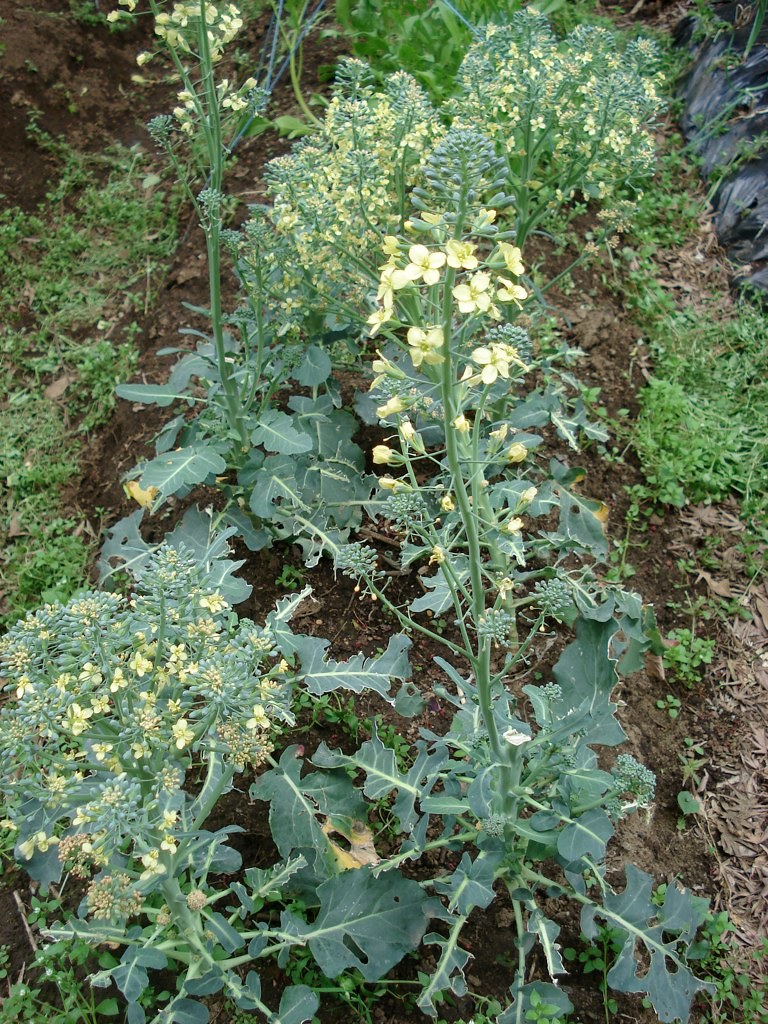This photograph captures a garden scene, bathed in natural light on what seems to be a sunny day. The garden features a mix of light and dark green plants, some of which are adorned with small yellow, four-petaled flowers clustered together. There is a noticeable trench or patch of dirt with a different texture and consistency, possibly indicating recent digging or a distinct planting area. The plants vary in size; some have large leaves and are growing upwards toward the light, while others are smaller but also flowering. Scattered across the brown dirt are patches of grass, weeds, or clover. The lighter soil on the right side indicates it has not been touched by rain, contrasting with the darker soil on the left. In the background and on the edges, dark green plants thrive, and the top right corner reveals what appears to be the edge of a tarp, contributing to a grayish-black area in the image. Overall, the garden seems to be flourishing with a variety of plants and blossoms, captured during daylight.